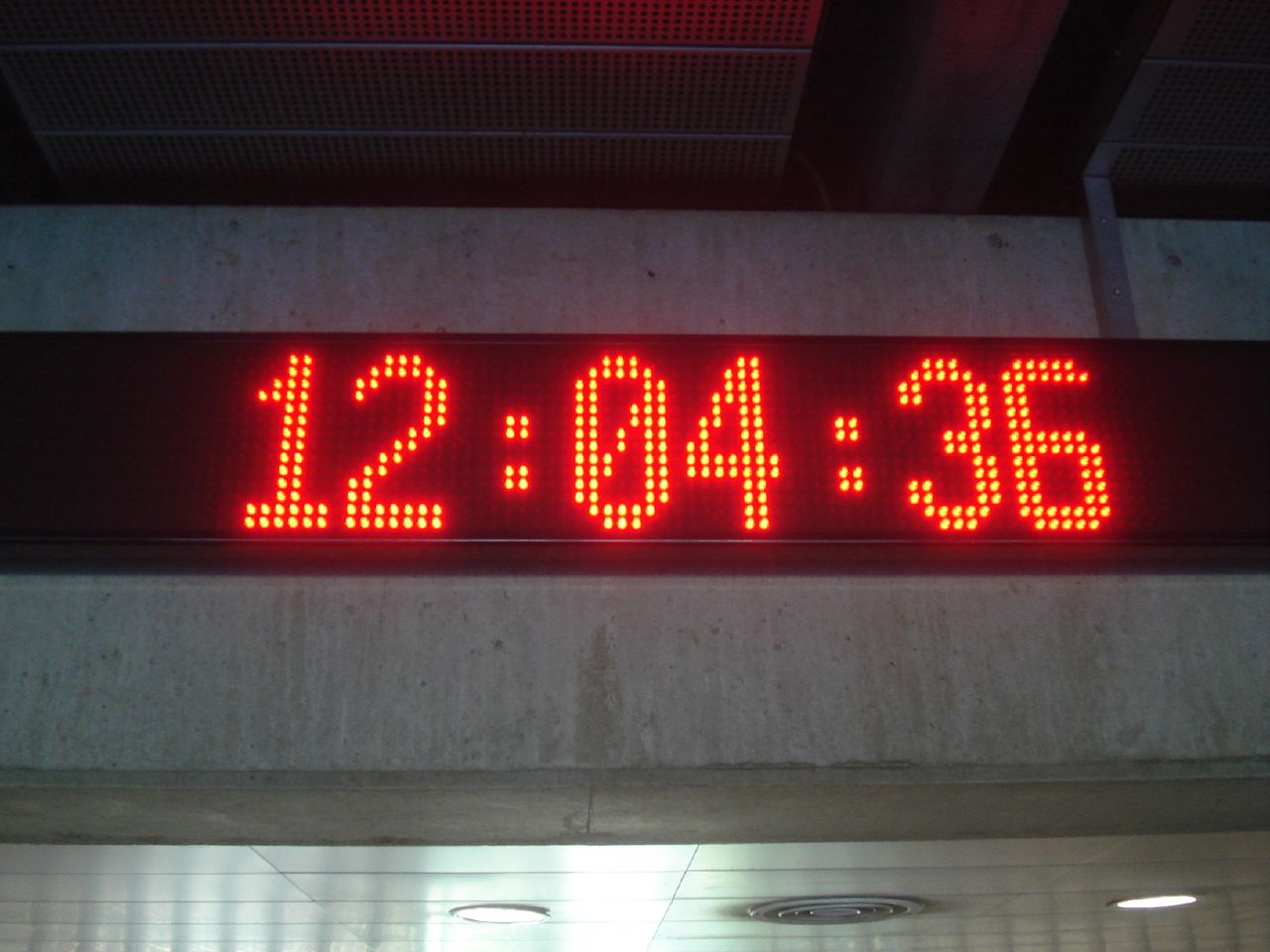The image features a tile ceiling at the very bottom, illuminated by a white light on the left and a red light on the right. Multiple circular objects, possibly smoke detectors, are affixed to the ceiling. At the top, there is a gray wall adorned with various LED dots displaying the time 12:04:36 in red. Additionally, clusters of small dots can be seen near the very top, suggesting either decorative elements or additional lighting. The wall itself appears to be constructed of stone or concrete.